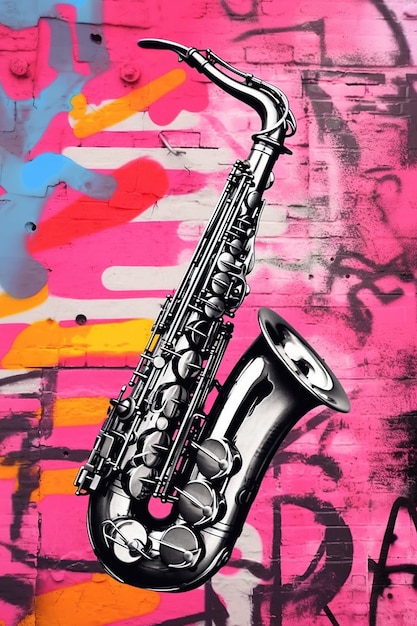This photograph presents a highly detailed silver saxophone, prominently positioned against a vivid, graffiti-adorned pink brick wall. The saxophone, depicted in black and white or possibly chrome, showcases an intricate array of shading and color variations that highlight its keys and buttons, numbering approximately eight to twelve. The background, predominantly pink, is a canvas of chaotic yet vibrant graffiti featuring an eclectic mix of colors including black, white, red, blue, orange, and yellow. The graffiti comprises random letters and abstract sprays, lacking specific words but adding to the dynamic visual appeal. Oriented in portrait format, the saxophone extends vertically, dominating the image with its striking contrast against the colorful, expressive mural behind it.